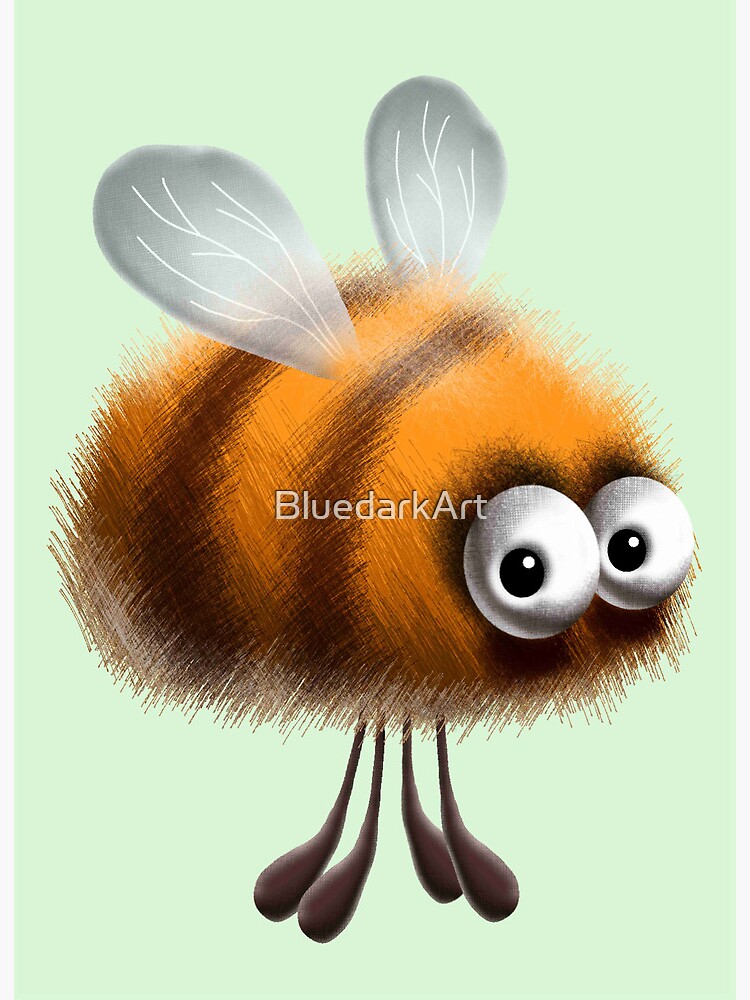The image features an artistic, cartoonish rendering of a bee on a light green background. The bee's body is round and puffy, colored orange with two dark brown stripes. Its eyes are large, white, and googly, directly positioned on the body since it does not have a distinct head. The bee has four thin, black legs hanging below that resemble golf clubs, and two small, translucent wings positioned on its back. The entire bee appears static, with no movement depicted. Across the center of the bee, the text "Blue Dark Art" is prominently displayed, presumably indicating the creator of the image. The overall appearance of the bee is cute and non-threatening, like a whimsical bumblebee.